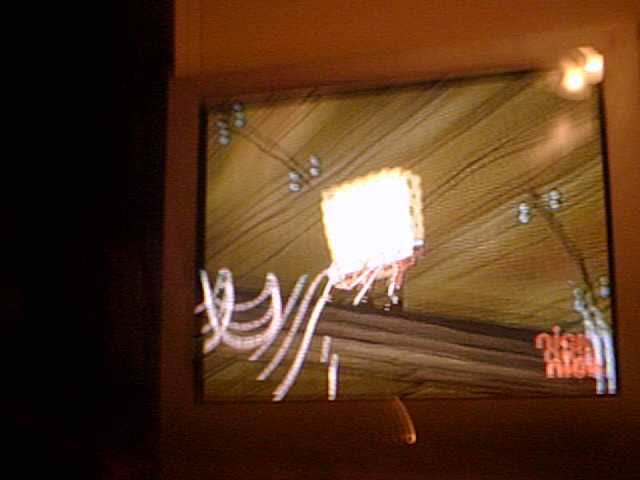In the image, we see a low-quality photograph capturing a flat-screen TV mounted on a wooden wall, which has a burnt orange or brown hue. The TV display showcases a dark scene from a Nick at Night TV show, featuring the character SpongeBob SquarePants at the center. The details of SpongeBob are partially obscured; his face is washed out and white due to the image's poor quality, but you can discern his black boots, square body, and brown pants. The TV screen also shows a wooden floor and some white lights that appear to be emanating from SpongeBob. Additionally, there are diagonal lines and small gray circles, possibly reflections or artifacts from the photograph. The overall lighting suggests the photo was taken in a dimly lit room, with the TV and a possible camera flash being the primary sources of light. The TV is supported by a sturdy wooden stand affixed to the wall.